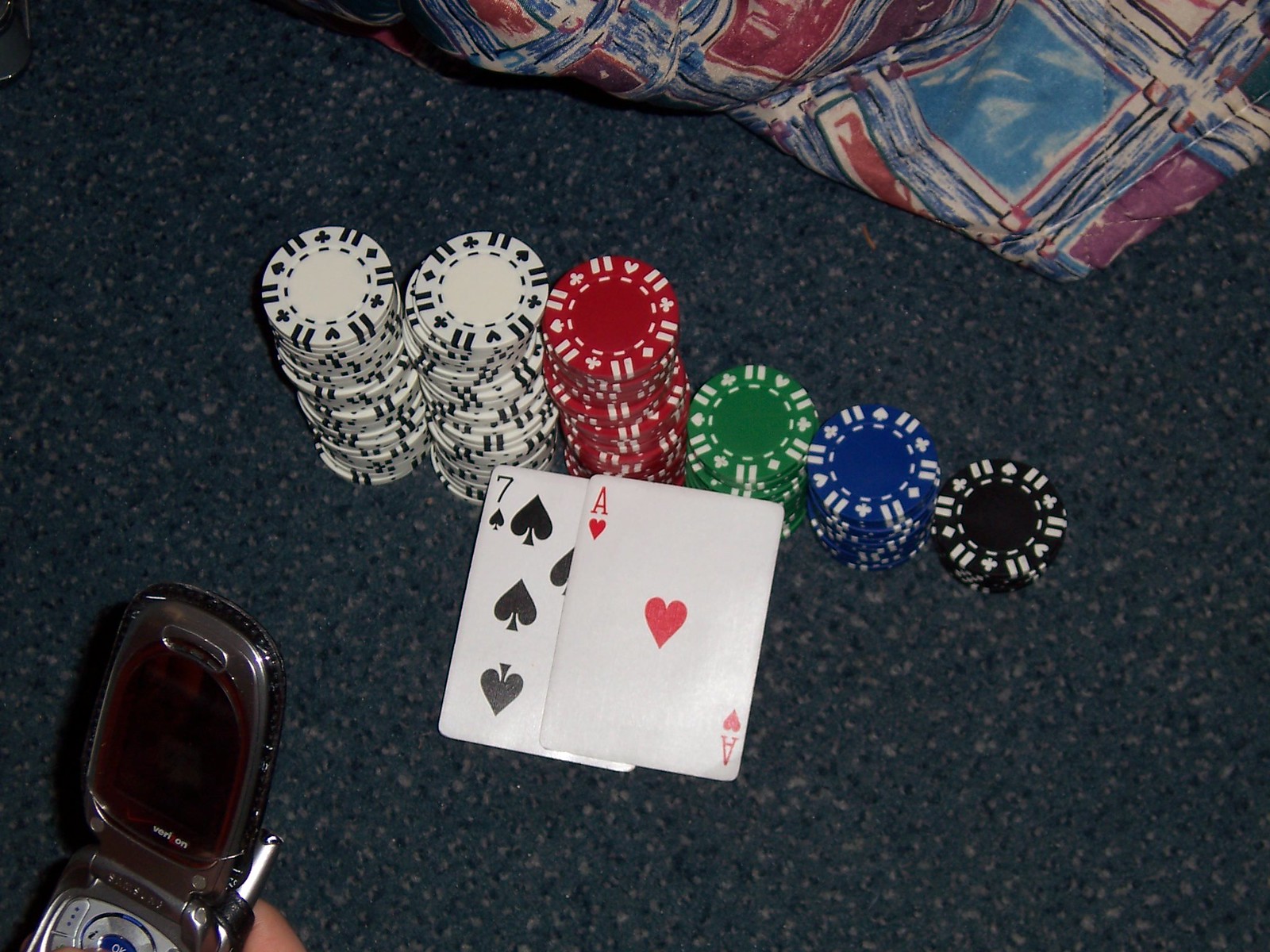In this top-down, first-person point of view image, it appears the scene is set on a blue felt surface, potentially a poker table or perhaps a carpeted floor that resembles an old rug. Arranged on this blue fabric are several neatly stacked poker chips. To the left, there are two stacks of white and black poker chips featuring the four suits: diamonds, spades, hearts, and clubs. Next to these, moving to the right, is a red stack followed by a smaller green stack. Continuing right, there's a dark blue stack and finally, a smaller black stack at the far right.

Adjacent to these poker chip stacks are two face-up playing cards: the seven of spades and the ace of hearts. In the bottom left corner of the image, a partial view of a hand, specifically a white-skinned finger, is visible holding an open flip phone displaying the Verizon symbol. At the very top of the image, there's a fabric with vibrant colors of blue, red, purple, and orange, evoking the impression of a child's drawing or colorful scribbles.